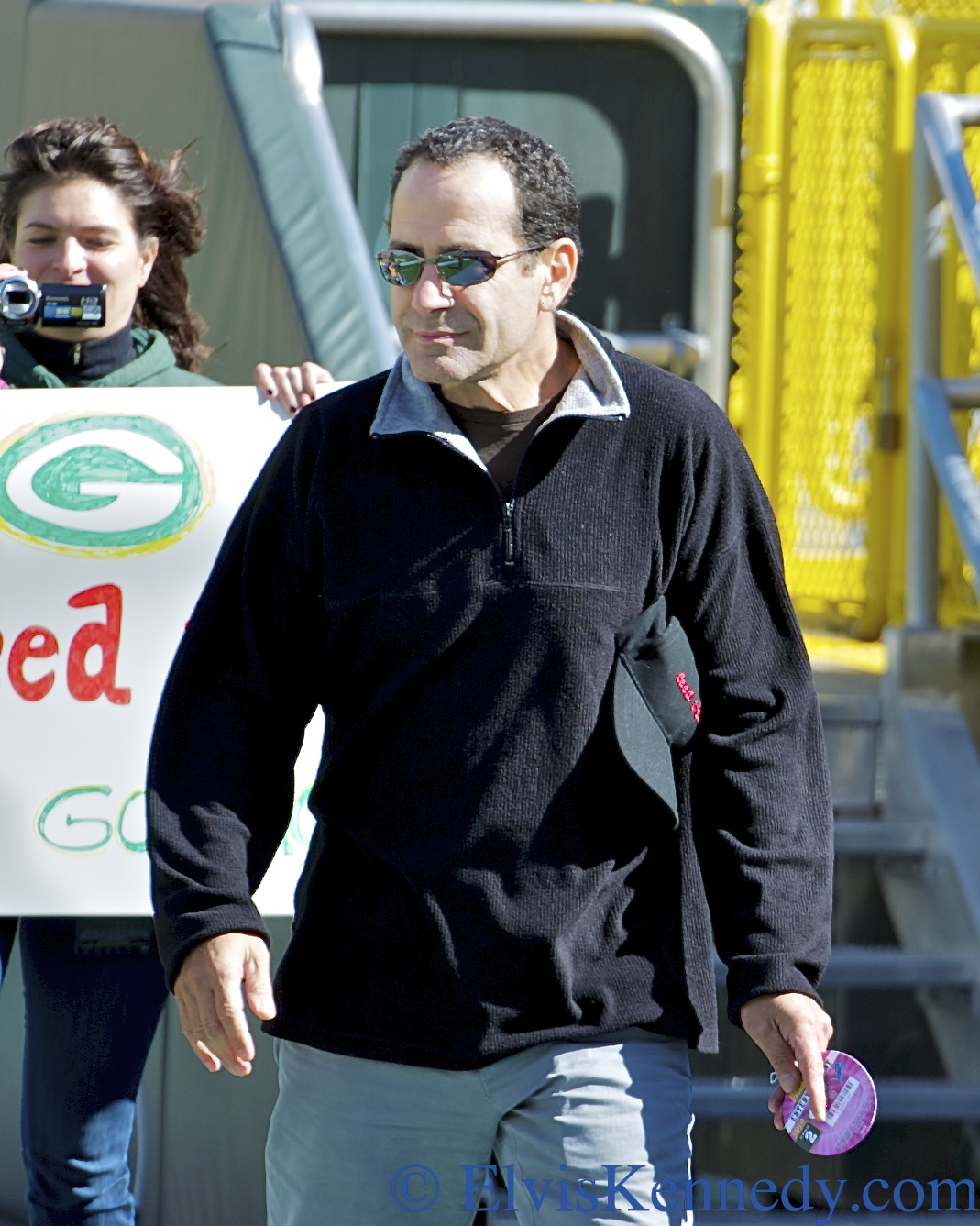The image showcases a man visible from his thighs up, wearing a long-sleeve dark blue corduroy zip-up sweatshirt over a greenish-brown t-shirt, light blue jeans, and small reflective sunglasses. He has short brown hair with noticeable balding and his head is tilted slightly to the left. In his right hand, he's holding a small disc with a purple spiral pattern on it. In the background to his left, a woman with brown hair holds a sign featuring red and green text. The scene appears to be outdoors, as there is a truck door visible behind the man. Additionally, the bottom right corner of the image contains a caption in dark blue font that reads "copyright ElvisKennedy.com".